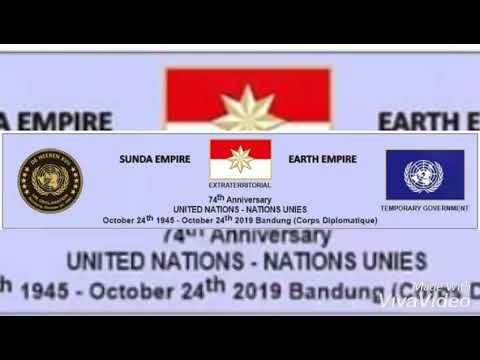The image is an informational graphic with a black header and footer, most likely a screen capture with a watermark that reads "Made with Viva Video." The central section of the graphic features a landscape-oriented, panoramic rectangle with a periwinkle blue background. On the left side, there's a round seal with a brown background and a gold or bronze globe at the center. This globe is encircled by laurel leaves and five stars on either side, along with a map of the world and feather motifs, and some blurry text that is hard to decipher.

In the center of this rectangle, there's a rectangular flag with a red upper half and a white lower half, featuring an eight-pointed white and gold star in the middle. Below this flag, the text reads, "Extra Historical" or possibly "Extraterritorial," followed by, "74th Anniversary United Nations, Nations Unis, October 24th, 1945 to October 24th, 2019, Bandung Corps Diplomatique."

To the right, there is another blue flag with a white logo similar to the one on the left, featuring a globe and laurel leaves, which is associated with the United Nations. Below this flag, it reads, "Temporary Government."

The background of the entire central section is an enlarged, slightly out-of-focus version of the same central banner, repeating the visual elements and text in a zoomed and pixelated manner.